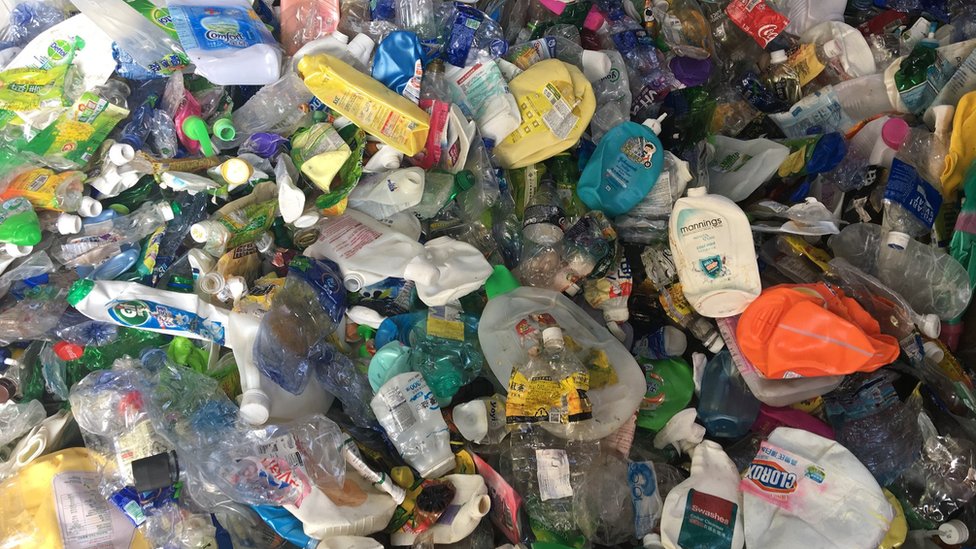The photograph depicts an overwhelming pile of discarded and crushed plastic items, predominantly consisting of a myriad of bottles and containers. These include various types of bottles: milk, water, juice, soda (notably Coca-Cola), and cleaning products like Clorox. The containers are assorted in colors, with some being transparent, blue, yellow, green, and more, featuring colorful caps that are mostly white, green, and pink. The image, taken from an overhead perspective, is densely packed, so much so that it leaves nothing else visible besides the plastic waste. In specific areas, such as the bottom right, a Clorox bottle and nearby green and orange containers can be identified. The top middle area is dotted with two yellow containers, while the bottom left showcases another yellow container with a white label. The entire scene emphasizes the chaotic jumble of recyclable plastics, reflecting a stark visual of environmental pollution.